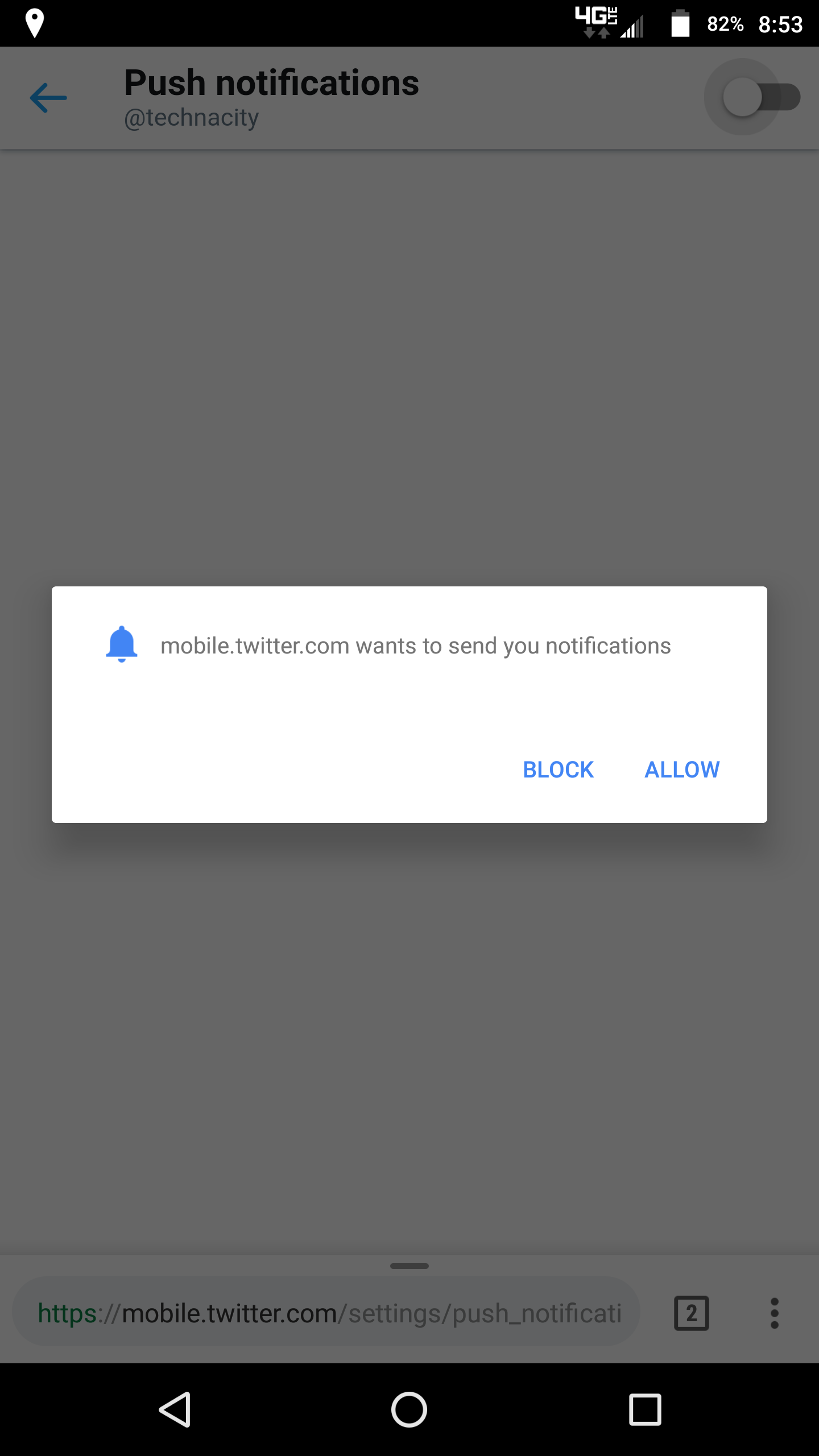This screenshot from a mobile device displays a Twitter settings page for push notifications. The top of the screen showcases a typical mobile status bar, indicating a 4G LTE connection with three out of five bars of signal strength and a battery level of 82%. The time shown is 8:53 AM. The device's screen is in light mode but dimmed due to an active pop-up window. At the top left, there is a blue back arrow. The page title reads "Push Notifications," followed by the user or page label "Technicity."

A prominent white pop-up window in the middle of the screen includes a blue notification bell icon and a message stating, “mobile.twitter.com wants to send you notifications.” The window presents two response options, "Block" and "Allow," both in blue font.

Below this pop-up, the URL displayed in the browser's address bar is "https://mobile.twitter.com/settings/push_notifications." Additional browser elements include two tabs, three vertical dots for more options, and at the bottom of the screen lies a navigation bar featuring, from left to right, a back arrow, a home circle, and a task view square.